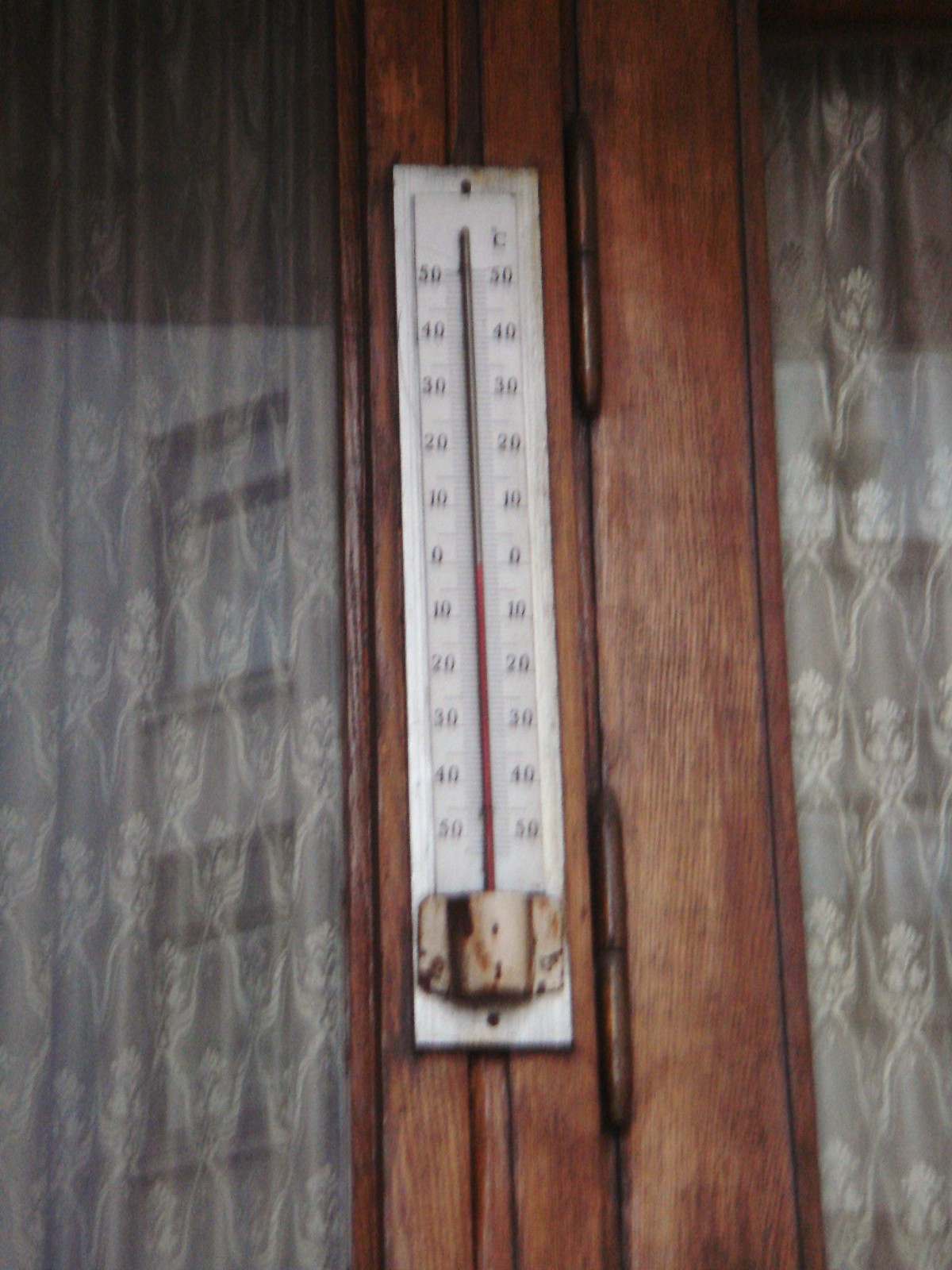The photograph captures a vintage thermometer mounted on the exterior surface of a door. The door, constructed from brown wood, features matching brown hinges and is flanked by glass panes on either side. These glass panes showcase delicate white lace curtains, suggesting a quaint and cozy interior behind the door. The thermometer, which appears to be made of metal, is installed vertically and shows signs of age, particularly rust spots at its lower end where the mercury resides. The device exclusively measures temperature in Celsius, with a scale ranging from 50 degrees above zero to below zero. Notably, there is no Fahrenheit scale present. Currently, the mercury indicates a temperature of zero degrees Celsius. This detailed glimpse of the weather instrument hints at its utilitarian heritage while blending seamlessly with the rustic charm of its surroundings.